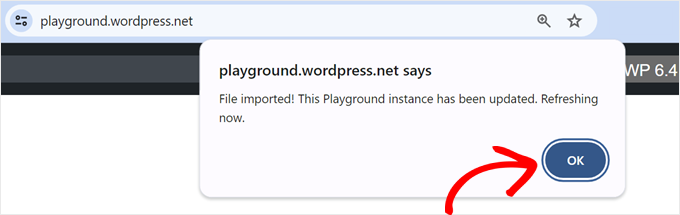**Detailed Caption:**

This image is a screenshot of a website, identifiable by the visible URL at the top left corner that reads "playground.wordpress.net". Adjacent to the URL, on the right, there are three icons: a magnifying glass with a plus symbol inside it, possibly indicating a zoom-in function, and a star, likely for bookmarking.

Just below this URL section, the text "playgroundwordpress.net" is repeated. Below this text, a notification states, "File imported. This playground instance has been updated. Refreshing now," signifying that a file has been successfully imported and the instance is in the process of refreshing. A red arrow curves from the bottom right towards an "OK" button, emphasizing that user action is needed to continue. The "OK" button itself is small, oval-shaped, with white text on it.

The background of the screenshot is mainly white at the bottom, with the pop-up notification overlaying part of the page content. In the top right corner, the text "WP 6.4" is displayed, suggesting that the website is running on version 6.4 of WordPress. Additionally, there is a filter button located at the top left, which features a pattern of circle-minus symbols, indicating potential filter options.

Overall, the screenshot implies that the user has completed an import task and needs to click "OK" for the changes to take effect, thus refreshing the page as part of the process.